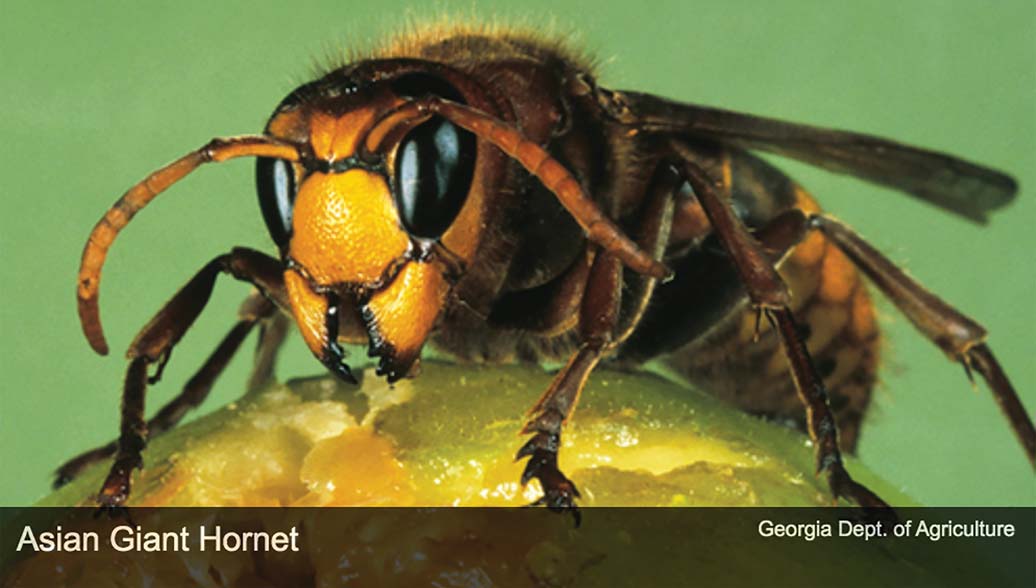This photograph presents a striking close-up of an Asian giant hornet, captured with a macro lens that reveals intricate details. The hornet, facing the camera, has large, oval, black eyes and yellow mandibles tipped in black. Its head is prominently yellow, complemented by yellow antennae and a brown furry abdomen with distinctive yellow and black stripes. The creature's brownish legs and body are easily distinguishable. With its wings folded neatly behind its back, the hornet is perched on what appears to be a round, yellow surface, possibly a piece of fruit. The setting features a light green background, enhancing the vivid colors of the hornet. At the bottom of the image, there's a translucent black triangular overlay with white text on either side. On the left, it reads "Asian Giant Hornet," and on the right, it states "Georgia Department of Agriculture." The photograph highlights the hornet in such clarity that every segment and hue, from yellow to lime and orange, is observed, making the intimidating aspect of this insect undeniably apparent.